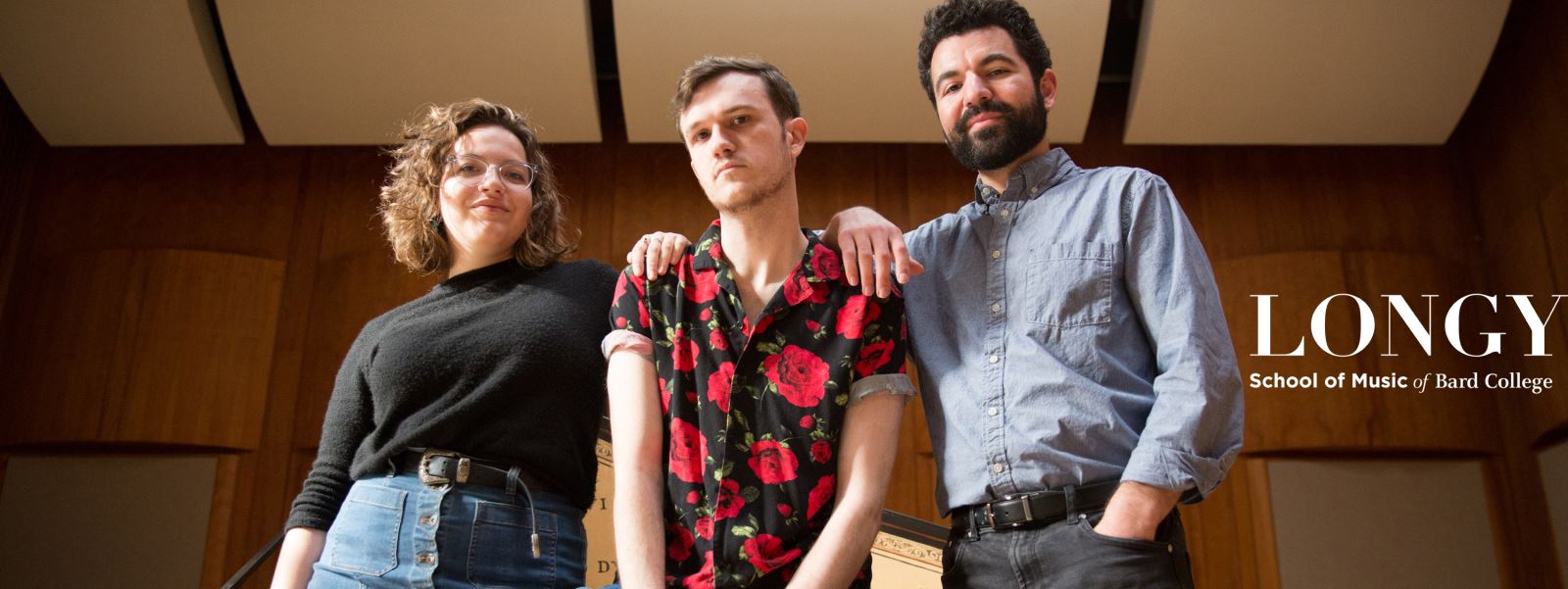This is a color photograph in landscape orientation, depicting three individuals set against a backdrop of a room with dark wood paneling and a white suspended ceiling, indicative of an acoustic room. On the right side of the image, in large white text, it reads "Longy," and below it, "School of Music of Bard College." The photograph captures the subjects from a low angle, creating the impression that they are looking downward at the viewer.

The woman on the left, approximately in her 40s or early 50s, has shoulder-length curly and wavy brown hair and is wearing glasses. She is dressed in a black turtleneck sweater with rolled-up sleeves, a black belt, and a jean skirt. Her expression is friendly as she smiles down at the viewer.

In the middle stands a younger man, around 22 years old, with short brown hair. He is dressed in a short-sleeved black button-up shirt adorned with red rose patterns and looks slightly impatient. His hands are resting on his sides, emphasizing his central position between the two older individuals.

On the right is an older man, also likely in his 40s or early 50s, of Hispanic descent, with black hair and a beard. He is wearing a long-sleeved navy blue collared shirt, paired with jeans and a black belt. His right hand is in his pocket, and he has a half smile as he looks down towards the viewer. Both he and the woman next to him have their hands placed on the shoulders of the young man in the center, creating a sense of connection and support among the trio.